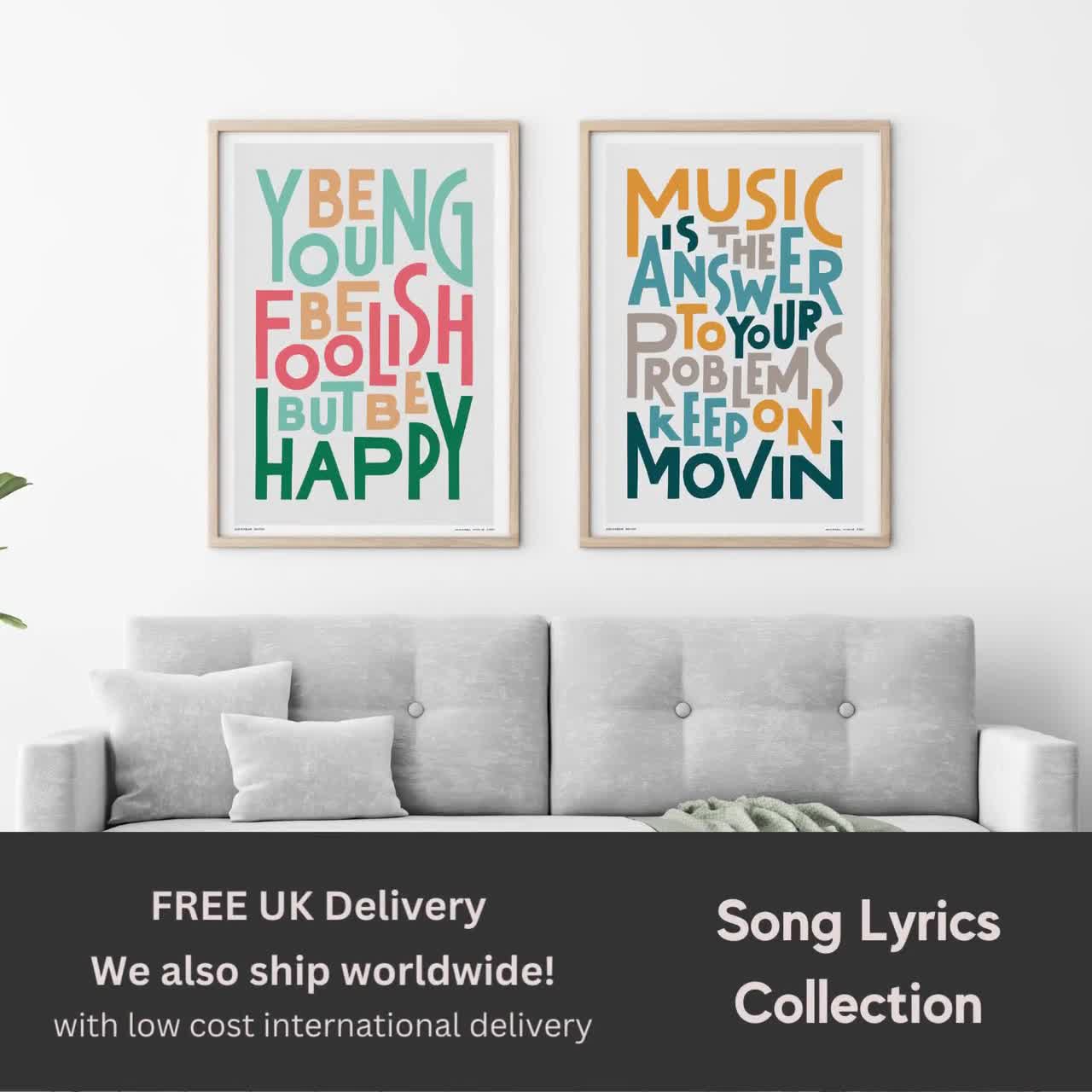The advertisement depicts a cozy, gray loveseat-style sofa adorned with a blanket draped on the right side and two throw pillows on the left. Above the loveseat hang two framed posters. The left poster features the phrase "Be young, be foolish, but be happy" in youthful, colorful fonts designed to appeal to a younger audience. The right poster reads "Music is the answer to your problems, keep on moving," making a strong artistic statement. The bottom of the image includes a banner advertising "Song Lyrics Collection" with a note about delivery options stating "free UK delivery" and "low cost international delivery."